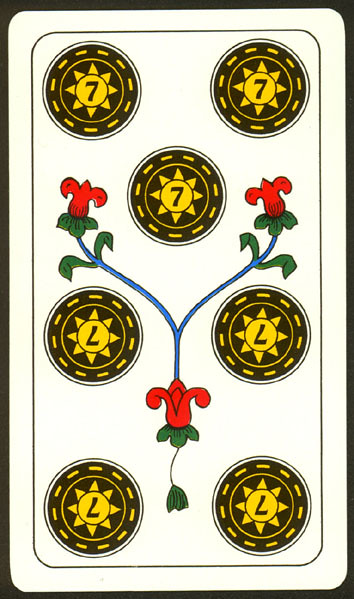This image displays a digital scan of a vertically oriented card, approximately the size of a playing card. The visible side features a complex pattern of seven concentric circular designs, each showcasing a meticulous arrangement of colors and shapes. 

Each circle is composed as follows:
1. **Outermost layer:** A thin black ring.
2. **Second layer:** A white band that separates the outermost ring from the next section.
3. **Third layer:** A broader black ring adorned with dashed yellow lines, resembling highway markings.
4. **Fourth layer:** Another thin concentric yellow ring.
5. **Innermost layer:** A black circle filled with a star pattern created by eight small triangles, arranged circumferentially.
6. **Central feature:** A bold black number "7" prominently displayed in the center of each complex circle design.

The amalgamation of these detailed geometric elements, coupled with the striking contrast of black and yellow colors, gives the card a highly intricate and visually engaging appearance.